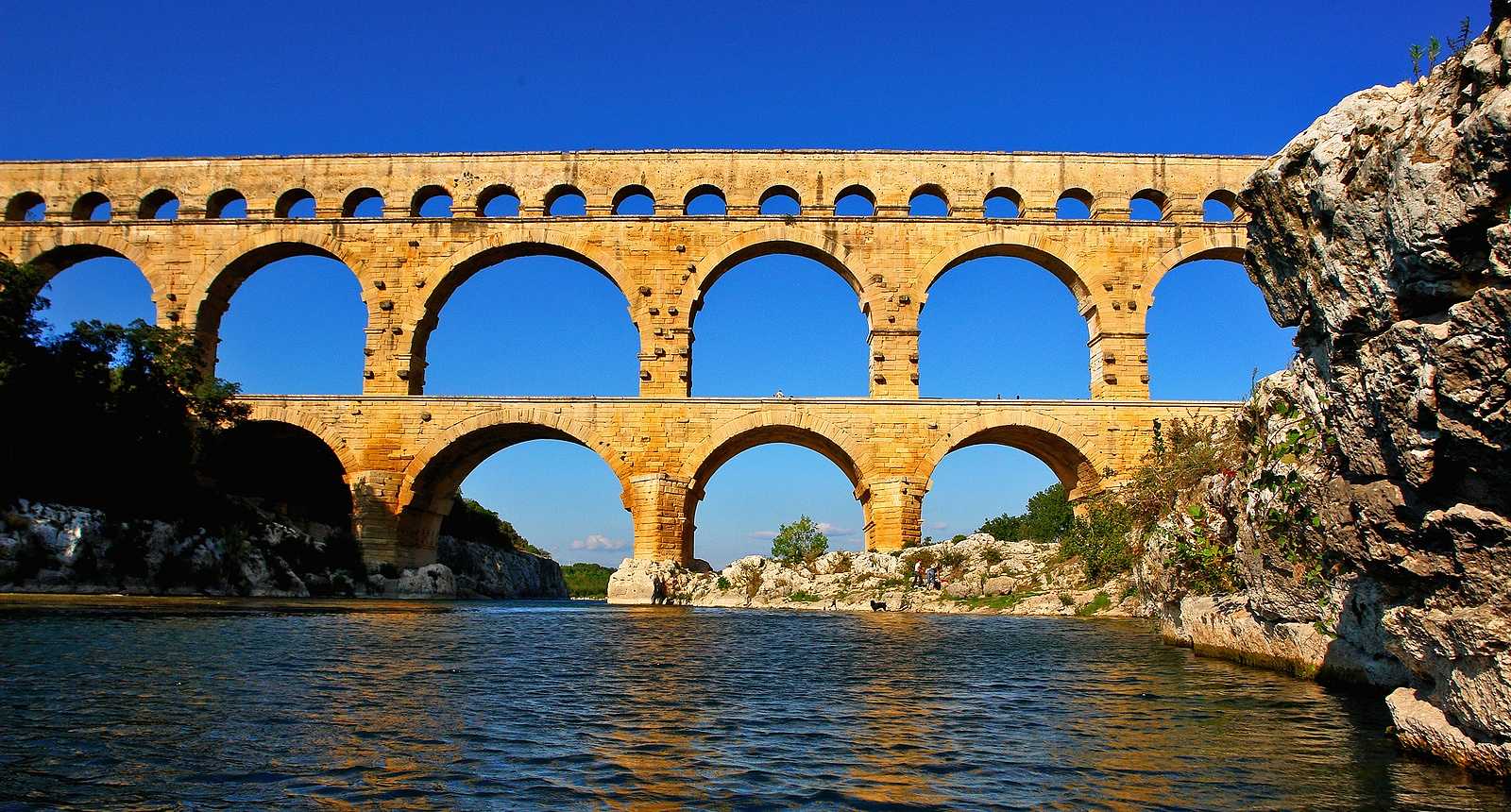This photograph captures the majestic Pont du Gard aqueduct in France, a historical marvel of Roman engineering. The expansive structure, built from stone, prominently features multiple tiers of arches with the middle tier being the most pronounced and the top tier consisting of smaller apertures. The aqueduct gracefully spans from a rocky cliff on the right to a tree-lined landscape on the left, bridging these distinct terrains over a wide, dark grey water body that reflects the impressive arches. The right side of the image showcases a rugged slope adorned with large, greyish-brown boulders beneath the aqueduct, where a couple of people and a dog can be seen. The water gently flows between the two land masses, enhancing the serene yet grandiose ambiance of the scene. The sky above is a clear blue, indicating the photo was taken during the day, providing a perfect backdrop to this awe-inspiring feat of ancient architecture.